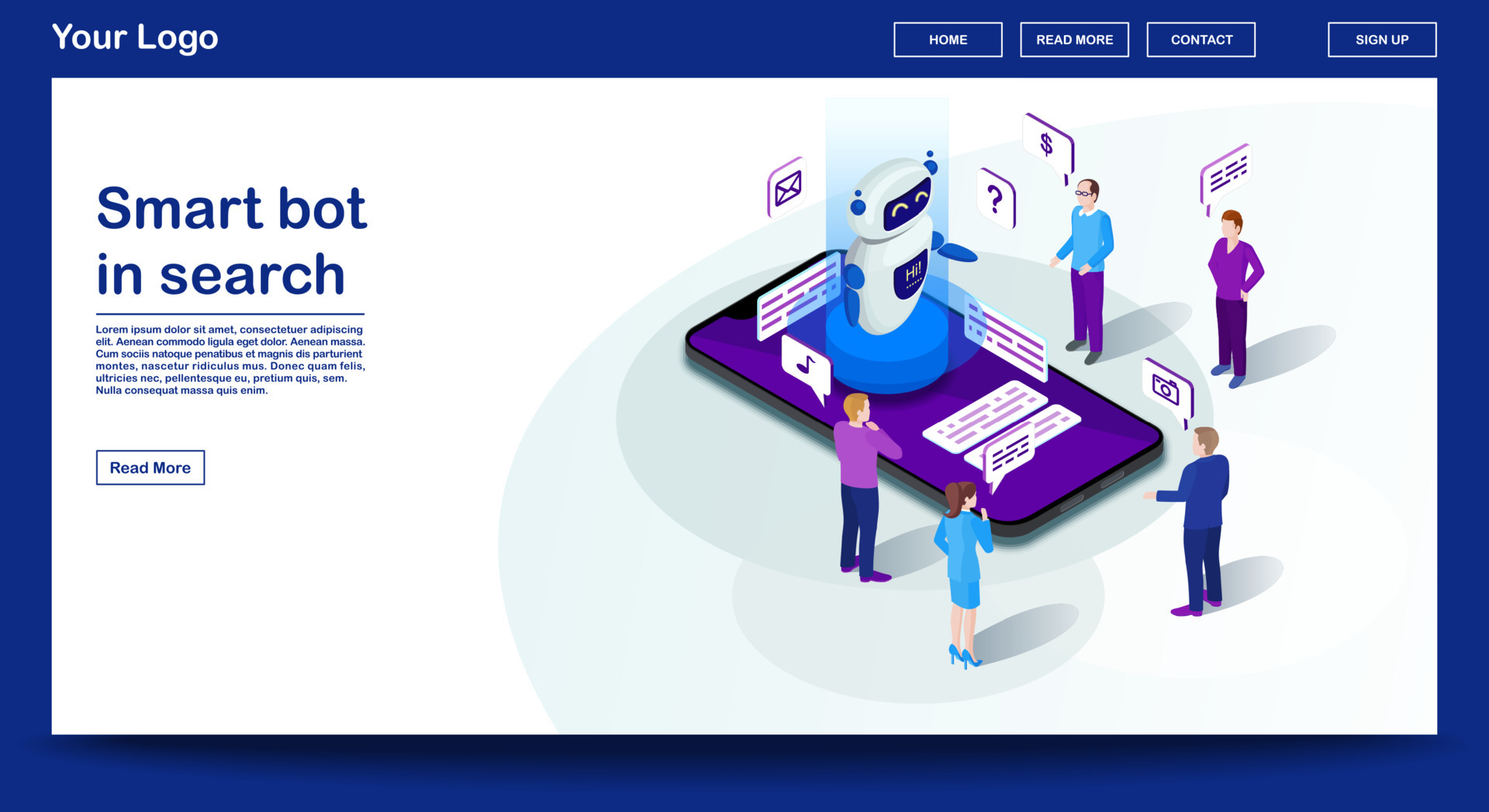This advertisement showcases a website with a sleek design and a dark blue border. In the upper left corner, white text reads "Your Logo" against the blue trim. The top right features four buttons in white text within white-outlined rectangles set against a blue background: "Home," "Read More," "Contact," and "Sign Up," slightly separated from the other three.

The main central area of the ad has a white background with green highlights and larger green circles towards the right. On the left, in the same blue as the border, the text reads "Smart Bot in Search." Beneath this title, a small, unreadable paragraph is separated by a line, with a blue-outlined white rectangle at the bottom saying "Read More."

Dominating the right side of the ad is an intricate, computer-animated scene. At its center is a robot on a rounded, purple rectangle platform akin to a smartphone. The robot, depicted as white with a black face, yellow eyebrows, and blue hands, stands in a holographic blue field. Surrounding the robot, five diverse cartoon characters—dressed in professional attire and sweaters—engage with it. The characters interact with various stylized symbols above them, including a music note, a dollar sign, a camera, an email icon, a question mark, and dashed lines representing text.

Overall, this detailed, multi-element advertisement effectively emphasizes the interactive and smart capabilities of the AI and highlights the website's navigational features.